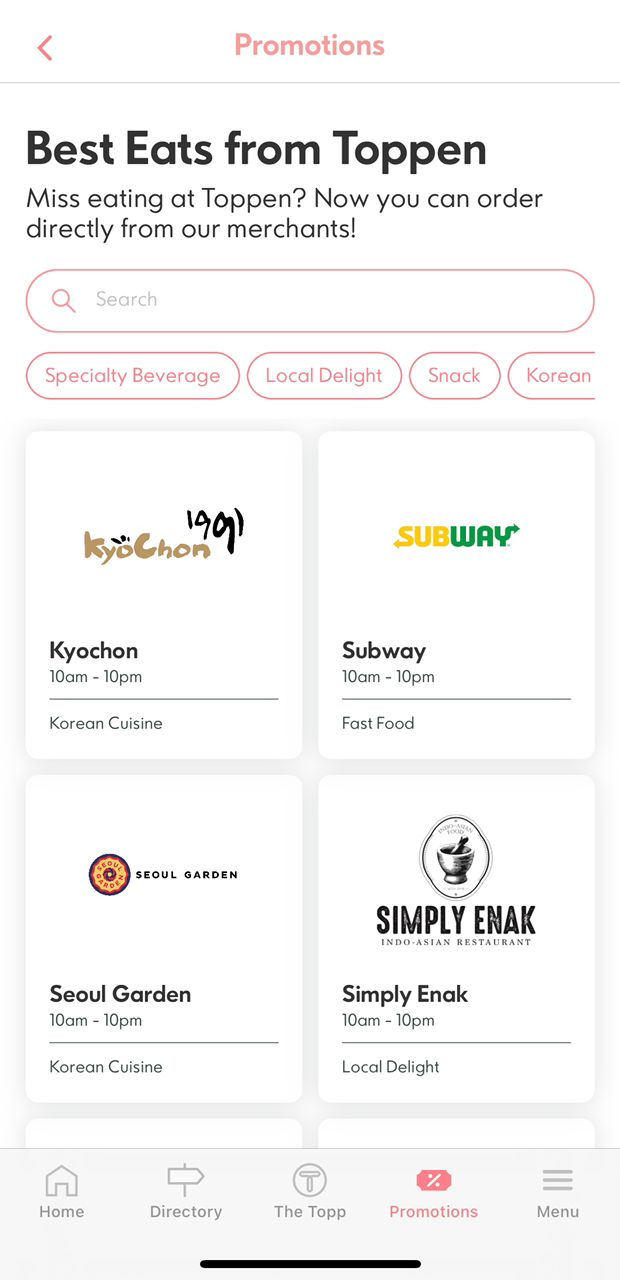The screenshot depicts a mobile interface, likely from a food ordering app. At the top center, in a pinkish hue, the word "Promotions" is prominently displayed. To the far left of this text, there is a back arrow, also in the same pink color. 

Below this, a thin gray horizontal line spans the screen. Directly underneath this line, in large bold black text, is "BEST EAT FROM TOPIN." Following this, in slightly smaller but still bold black font, it reads, "Best eating at Topin. Now you can order directly from our merchants."

Further down, there is a search field, accompanied by a series of filter options. These options include "Specialty Beverage," "Local Delight," "Snack," and "Korean."

Beneath the filter options, the screen is divided into four tiles. Each tile has a white background and features the logo of a different company in the center. The upper-left tile showcases "KyoChon," the upper-right displays "Subway," the lower-left highlights "Seoul Garden," and the lower-right features "Simply Enak." Each tile also includes the company's name, hours of operation, and type of cuisine at the bottom.

At the very bottom of the screenshot, the typical smartphone menu options are visible. From left to right, these include Home (symbolized by a house icon), Directory (indicated by a signpost icon pointing right), The Top (represented by a circle with a "T" inside), Promotions (highlighted in pink, matching the text at the top), and Menu (depicted by three parallel lines). The Promotions icon is notably in pink, signifying that it is the currently selected option, whereas the other icons are grey.